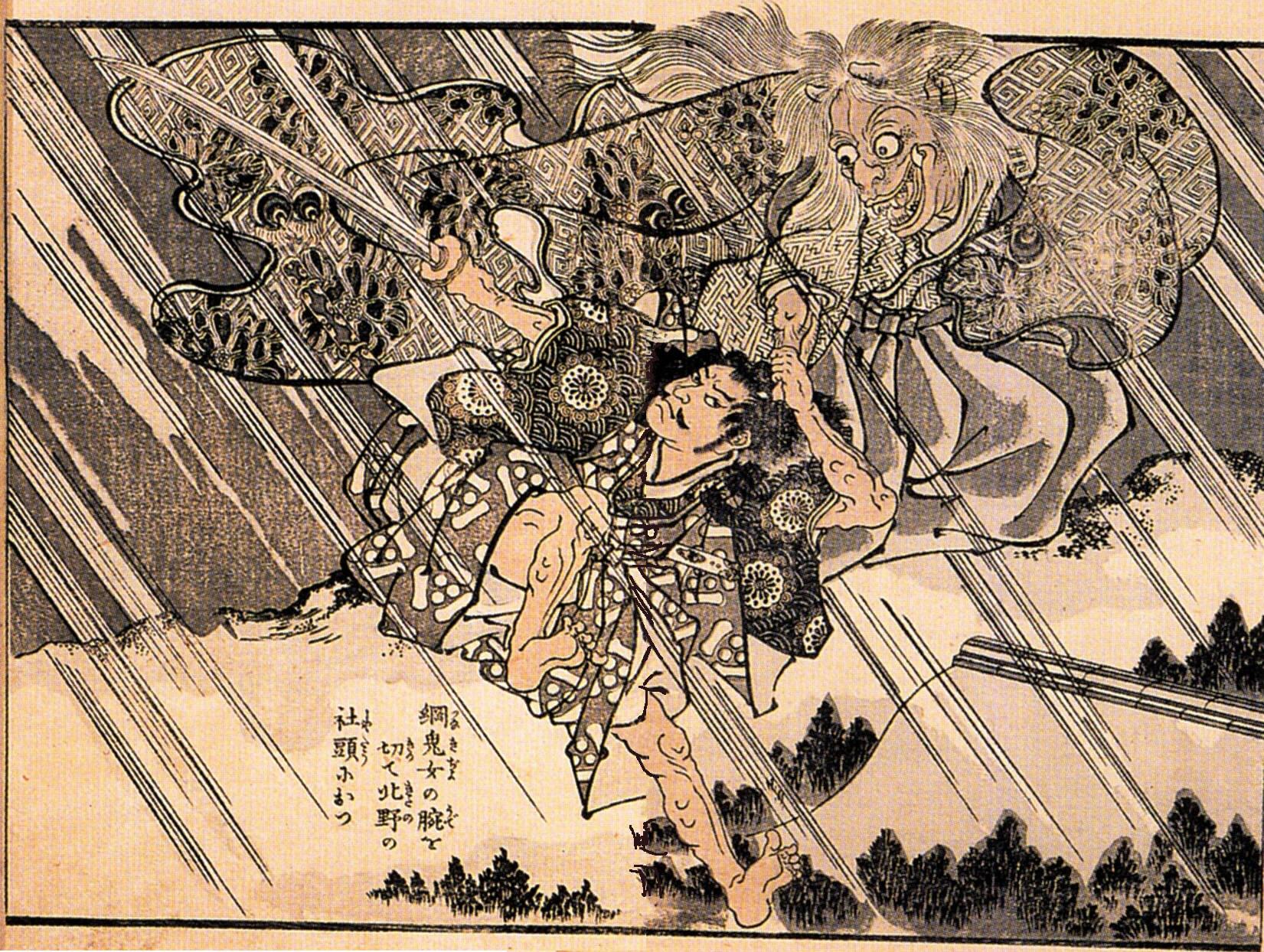This artwork seems to be a Japanese-style drawing done in sepia tones of beige, tan, black, and white. At its center is a man, possibly a warrior or fighter, dressed in a culturally intricate gown adorned with floral patterns, his long black hair flowing. He is captured in a dynamic, almost precarious, pose on one leg, brandishing a sword in his right hand. His facial features include a handlebar mustache. Above him floats an older man or demonic creature, depicted with a wild expression, big eyes, an open mouth showcasing a fang, and wearing a similar intricate gown. This figure appears to be engaged in combat with the man below.

The background features an earthy landscape with small tufts of trees or plants, mountain-like structures, and a mix of grass and rocks. There are also white streaks diagonally crossing from the top left to the bottom right, adding a dynamic and dramatic effect to the depiction. Asian script is noted towards the left-hand side, adding context and perhaps narrating an aspect of Japanese folklore or historical battle. The swirling light and dark patterns at the top create a sense of movement and tension between the two figures.